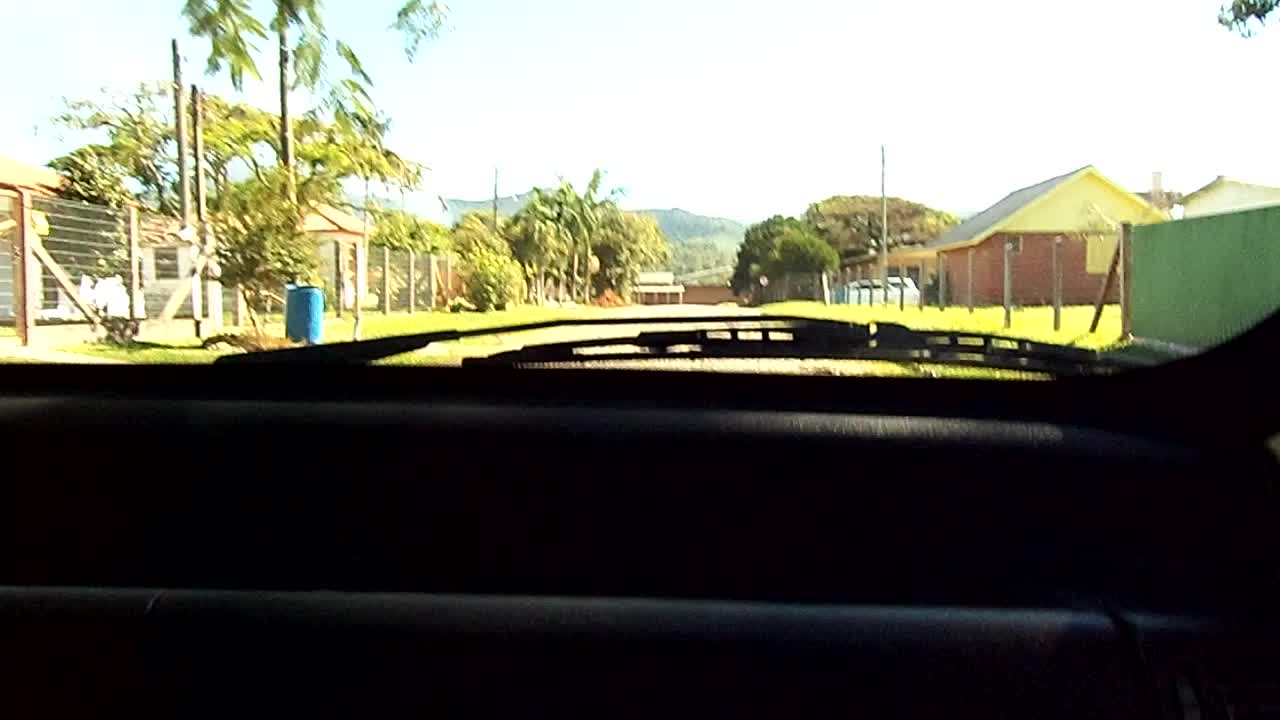A photograph taken from the interior of a car captures a serene countryside scene through the windshield, framed by the car's black dashboard and a visible windshield wiper. To the left, a tall palm tree stands alongside several low beige houses, each enclosed by high wire fences. A blue garbage can is placed by the roadside beneath another tree, contributing to the rustic ambiance. The backdrop features a range of distant mountains, partially shrouded by a line of trees that add depth to the landscape. On the right side, another segment of the wire fence reveals a brown brick house with a distinct white roof. In front of this house, a partially visible green fence is discernible, alongside a white car parked in the driveway. The setting exudes a peaceful, rural charm, underscored by the natural elements and scattered residences.